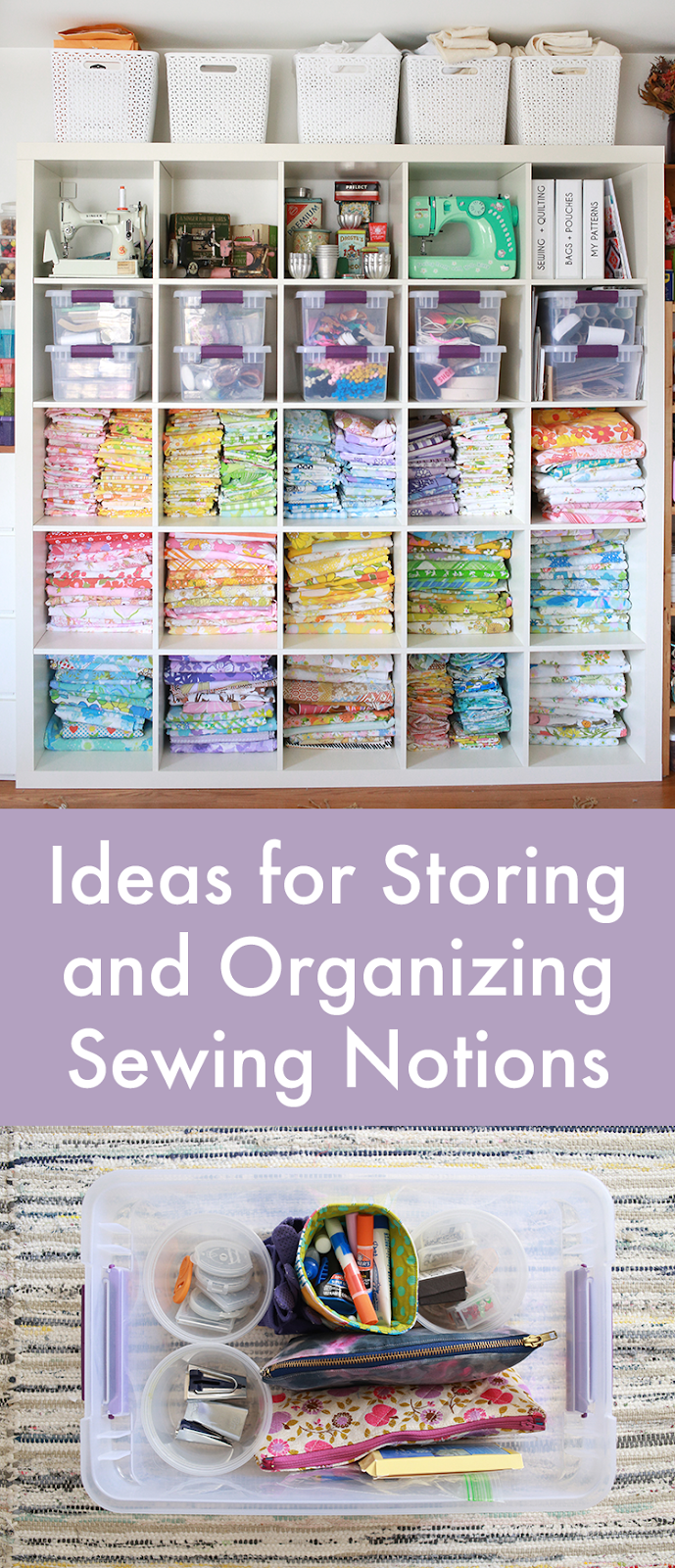This photograph depicts a highly organized and visually appealing poster, likely styled for a blog or Pinterest. The central focus of the poster is a text in white lettering on a light purple background that reads, "Ideas for Storing and Organizing Sewing Notions." Above this text, an extensive storage setup is showcased—a five-by-five shelf unit filled with a variety of colorful fabrics, small books, multiple sewing machines, and numerous translucent and white linen boxes containing threads, needles, and other sewing supplies. The overall aesthetic is clean, modern, and very organized, suggesting the creator is deeply invested in sewing, possibly as a profession or serious hobby. The bottom part of the image features an overhead view of a plastic storage bin, meticulously organized with small round cups, colorful sewing tools, and zippered bags, contributing to the busy and vibrant pastel color scheme of the poster.